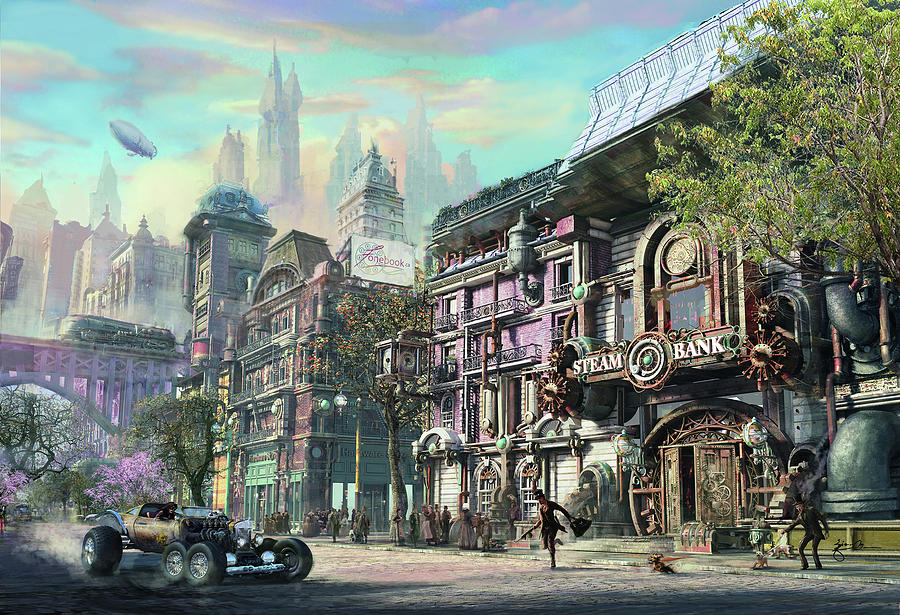This computer-generated artwork depicts an elaborate steampunk cityscape blending elements of both futuristic and Victorian-era design. Dominating the right side of the image is a building labeled "Steam Bank," adorned with pipes, tubes, and an intricate steampunk watch mechanism. In an action-packed scene, a man is seen running out of the Steam Bank, clutching a bag and brandishing a rifle, suggesting a bank robbery. His destination is a peculiar, brown, gear-laden vehicle parked across the street, with a woman seated in the passenger seat, ready to make a swift getaway.

The streets are bustling with people dressed in Victorian-era attire, including a man holding a dog with another dog chasing after the fleeing robber. The cityscape is dotted with towering buildings that stretch thousands of feet into the sky. In the background, a futuristic steam-powered train traverses a bridge surrounded by tall buildings and lush trees.

Above, a blue sky speckled with fluffy white clouds hosts various aerial craft, including a blimp or zeppelin on the left-hand side. The left side of the image also features a bridge with vibrant purple trees and illuminated by purple lights. Overall, the scene is rich with steampunk aesthetics, blending old-world charm with futuristic technology.